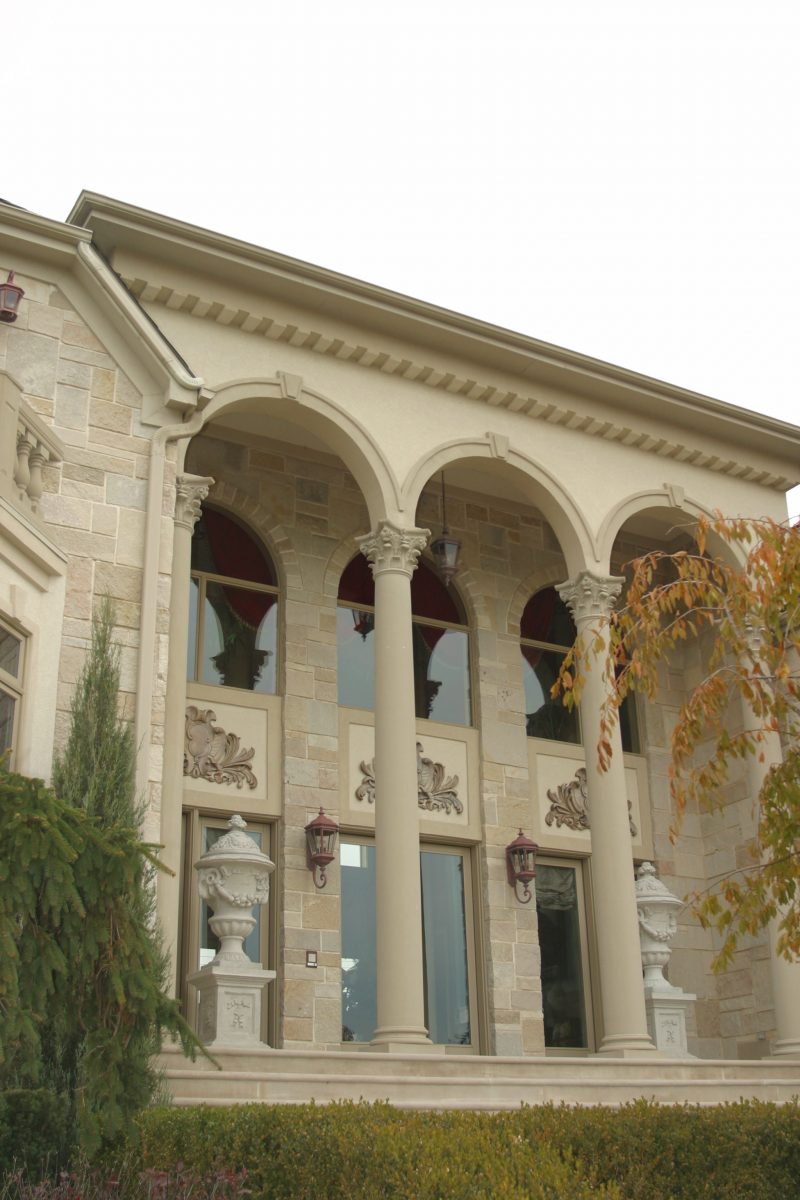This image features a grand stone building adorned with imposing, plastered columns leading up to a flat roof. Flanking the entrance are two large, ornate replicas of ancient Roman-style goblets, each mounted on substantial square pedestals. The building showcases a grand entrance with expansive glass doors, and balconies positioned on both the left and right sides of the facade. Above the entryway, three intricately designed elements reminiscent of decorative pieces often seen on festive tables, such as those used for Thanksgiving, add to the building's elegance. Additional windows are located above these decorative elements. In the foreground, a tree on the left side, along with some shrubbery and overgrown grass, contribute to the stately yet slightly untamed ambiance of the scene.